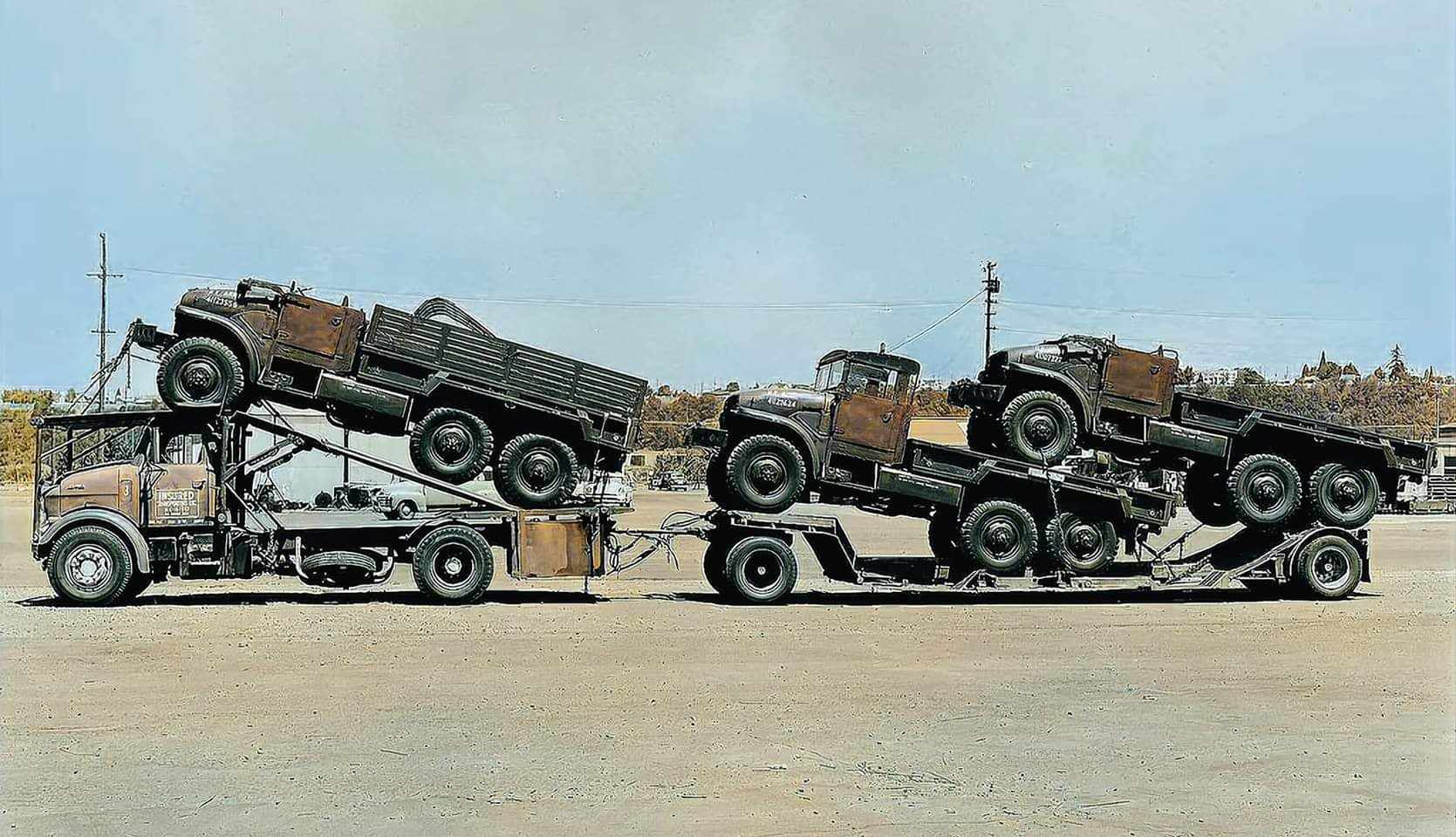The photograph depicts a large, 16-wheel, heavy-duty trailer towing three 12-wheel utility trucks in a barren, desert-like setting. All trucks are painted mostly black with brown doors, and are oriented to the left in a side view. The first truck features a spare tire hanging on its right side, and the remaining two are loaded on a flatbed trailer attached to it. The scene has a bright, sunny atmosphere, with a clear blue sky, some white clouds, and distant power lines overhead. The ground appears to be packed-down dirt or cleared sand, with minimal vegetation and some distant trees and hills providing a subtle backdrop. The image lacks any visible text, emphasizing the robust and sturdy configuration of the trucks in the otherwise stark environment.